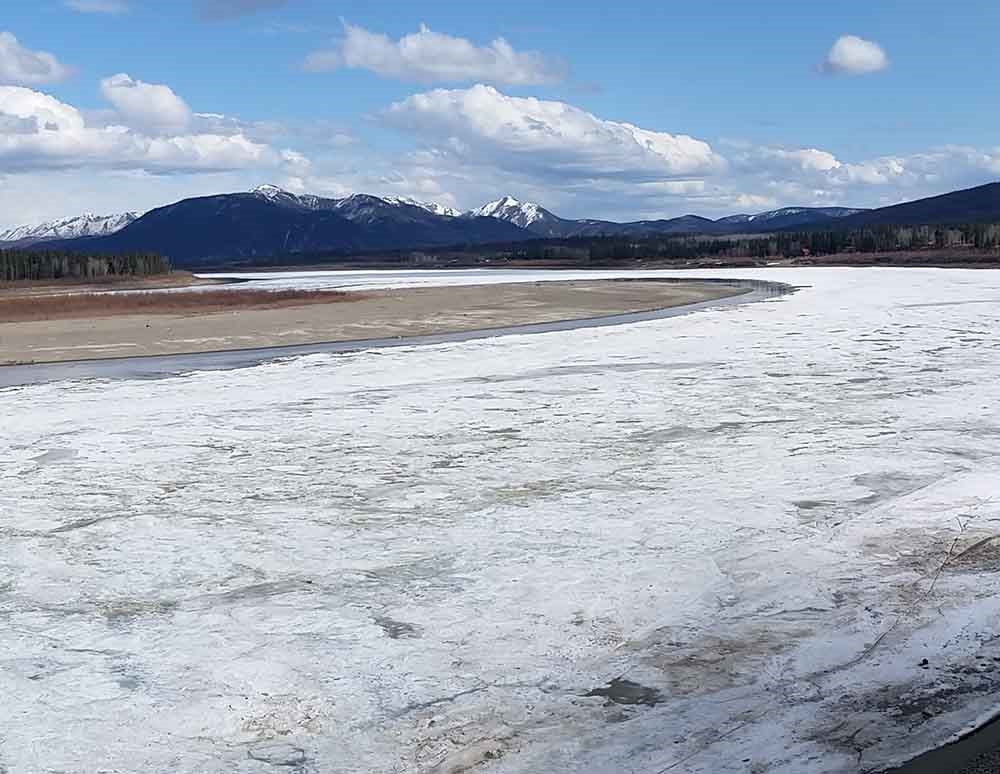This image is a stunning landscape photograph of the Alaskan wilderness, focusing on the frozen Yukon River. The river, dominated by a thick sheet of white ice with visible cracks, stretches across the lower portion of the square photograph. On the far bank, the barren, dark beige sand gives way to a stand of trees. The river winds off towards the left, enveloping the serene, mostly clear horizon.

Dominating the background are majestic, snow-capped mountain ranges. A particularly tall peak stands prominently in the center, flanked by lower mountain ranges that extend across the horizon. The mountains are a mix of snow-covered and bare dark areas, creating a striking contrast.

Above, the vast expanse of the sky is a clear, vibrant blue adorned with patches of white cumulus clouds. The clouds have bright upper portions lit by sunlight, while their lower sections remain in shadow, stretching from one end of the horizon to the other. This beautiful natural environment is a part of a study on the impacts of climate change in Alaska, showcasing the pristine yet changing wilderness.